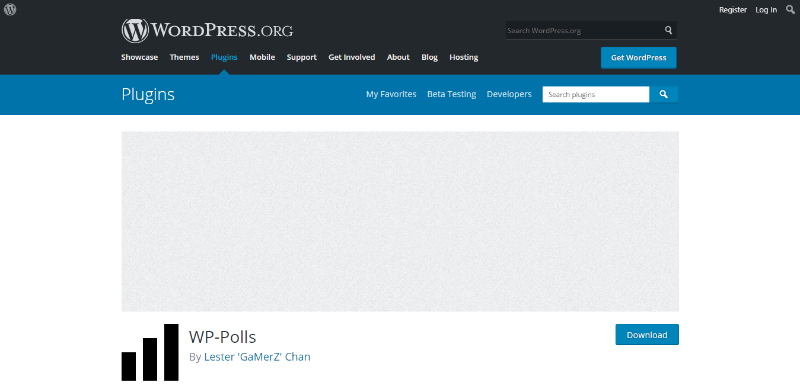**Screenshot of WordPress.org Desktop Website**

The screenshot captures the WordPress.org website in desktop orientation, showcasing its top header in a sleek carbon black color. Below the header is a blue navigation bar dedicated to plugins, prominently displaying "WordPress.org" at the top without a typical navigation bar. The full-screened webpage foregrounds the top menu with options including Showcase, Themes, Plugins (which is currently selected), Mobile, Support, Get Involved, About, Blog, and Hosting.

Positioned above the main content area are a search bar and a button labeled "Get WordPress." On the top right corner, options for 'Register', 'Login', and an additional search button are neatly aligned.

Directly beneath the highlighted plugins menu, there is a secondary plugins bar featuring categories such as My Favorites, Beta Testing, Developers, and Search Plugins. The sole plugin option displayed here is 'WP-Polls' by Lester Gamers (stylized as Lester Gamers with a "z-chan"). Next to the WP-Polls title is a graphical icon representing a graph with three black bars, currently unenabled. Accompanying this plugin entry is a download button, providing a direct call to action.